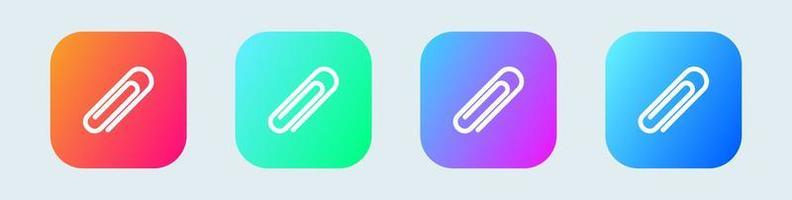The image is a horizontally rectangular graphic design with no border, featuring a light gray background. It showcases four rounded-corner squares, each containing a bold, white paperclip centered inside. The paperclips are diagonal, slanting to the right. From left to right, the squares are colored as follows: the first square transitions from a faded orange at the top left to red at the bottom right; the second square shifts from green at the top left to teal at the bottom right; the third square blends from light blue at the top left to light purple at the bottom right; and the fourth square gradients from lighter blue at the top left to darker blue at the bottom right. The image contains no text or additional elements.